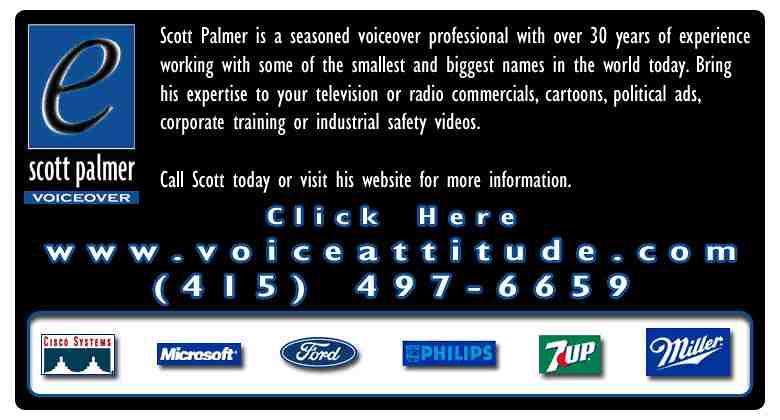The advertisement features a dark, possibly blue, landscape-oriented rectangular background. In the upper left corner, there is a logo consisting of a blue square with a black letter "E" inside it. Directly beneath the logo, the text "Scott Palmer Voiceover" is displayed in white.

Centrally positioned at the top is detailed text introducing Scott Palmer as a seasoned voiceover professional with over 30 years of experience. It elaborates on his extensive work with a range of clients, both small and large, and highlights his capability to lend his voice to television and radio commercials, cartoons, political ads, corporate training, and industrial safety videos. 

Further inviting potential clients to reach out, the text advises to "Call Scott today or visit his website for more information." The contact details include a call-to-action link "click here www.voiceattitude.com" followed by the phone number "415-497-6659."

Below this informative text, a series of logos from companies such as Cisco Systems, Microsoft, Ford, Philips, 7-Up, and Miller, are displayed, suggesting his collaboration or association with these reputable brands. The overall design resembles an electronic business card or digital flyer, effectively summarizing Scott Palmer's expertise and contact information.